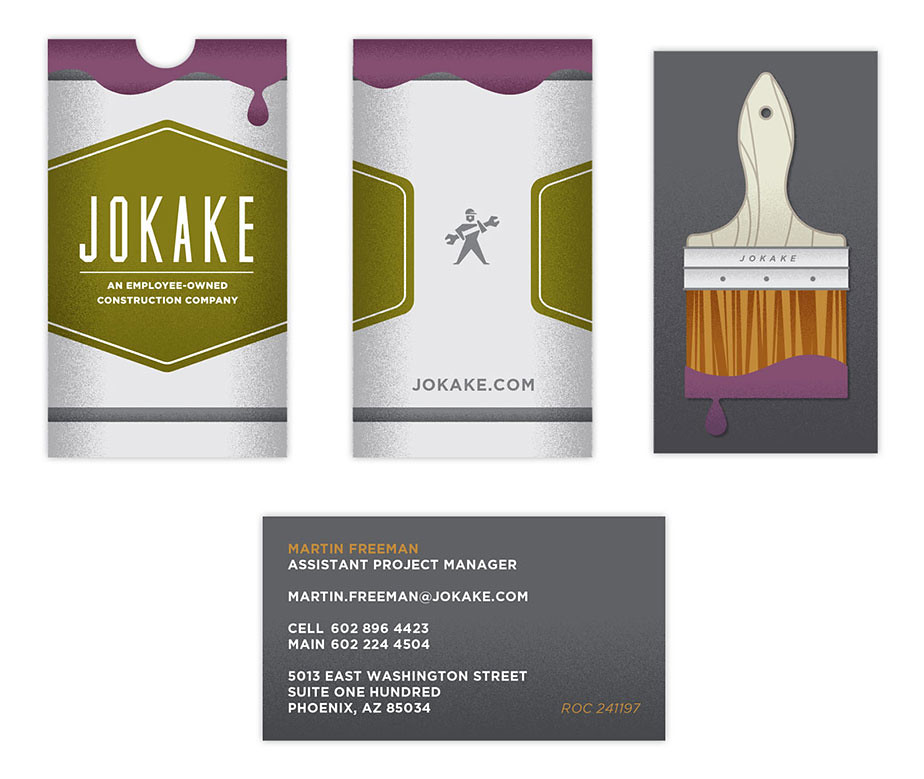This image is a detailed, color-illustrated business card comprised of multiple segments in a landscape orientation, integrating both graphic design and typography. The top half features three vertical portrait illustrations.

- The left segment displays the word "Jokake," spelled out as J-O-K-A-K-E in white letters against an olive-green, triangular background. Above this is a notched strip of purple that appears to be dripping paint, adding a dynamic and artistic touch. Beneath the company name, in smaller white font, the text reads, "An Employee-Owned Construction Company."

- The central segment continues this theme, showing a gray stick figure holding a wrench between two green ends, with the word "jokake.com" underneath. This part also has a similar purple paint design at the top and silver body that matches the overall aesthetic.

- The right segment is an illustration of a paintbrush with purple paint dripping from the bristles. The handle is detailed with the word "Jokake" imprinted on the aluminum strip attaching the bristles.

At the bottom of the image, there's a business card layout with a gray background. Highlighted in gold text at the top is the name "Martin Freeman," followed by white text that includes the title "Assistant Project Manager," an email address "martinfreeman@jokake.com," a phone number, and an address. The entire composition blends illustration, graphic design, and professional typography to create an engaging and informative business card.